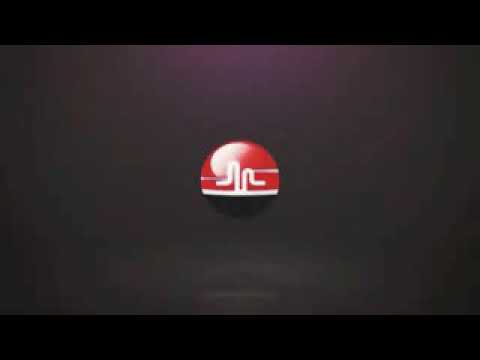The image features a circular disc centrally positioned against a blurred, gradient background comprising varying shades of maroon, black, dark gray, and purple. The backdrop is low-resolution, augmenting the image's abstract quality. The disc in the center is a graphical logo with its top three-quarters in vivid red, intersected by a white squiggle line. A horizontal white stripe also runs along the disc's bottom third, beneath which lies a black semicircle defining the bottom portion of the disc. The entire composition is framed within a horizontal 16 by 9 aspect ratio, bounded by black bars on the top and bottom, enhancing the landscape orientation.